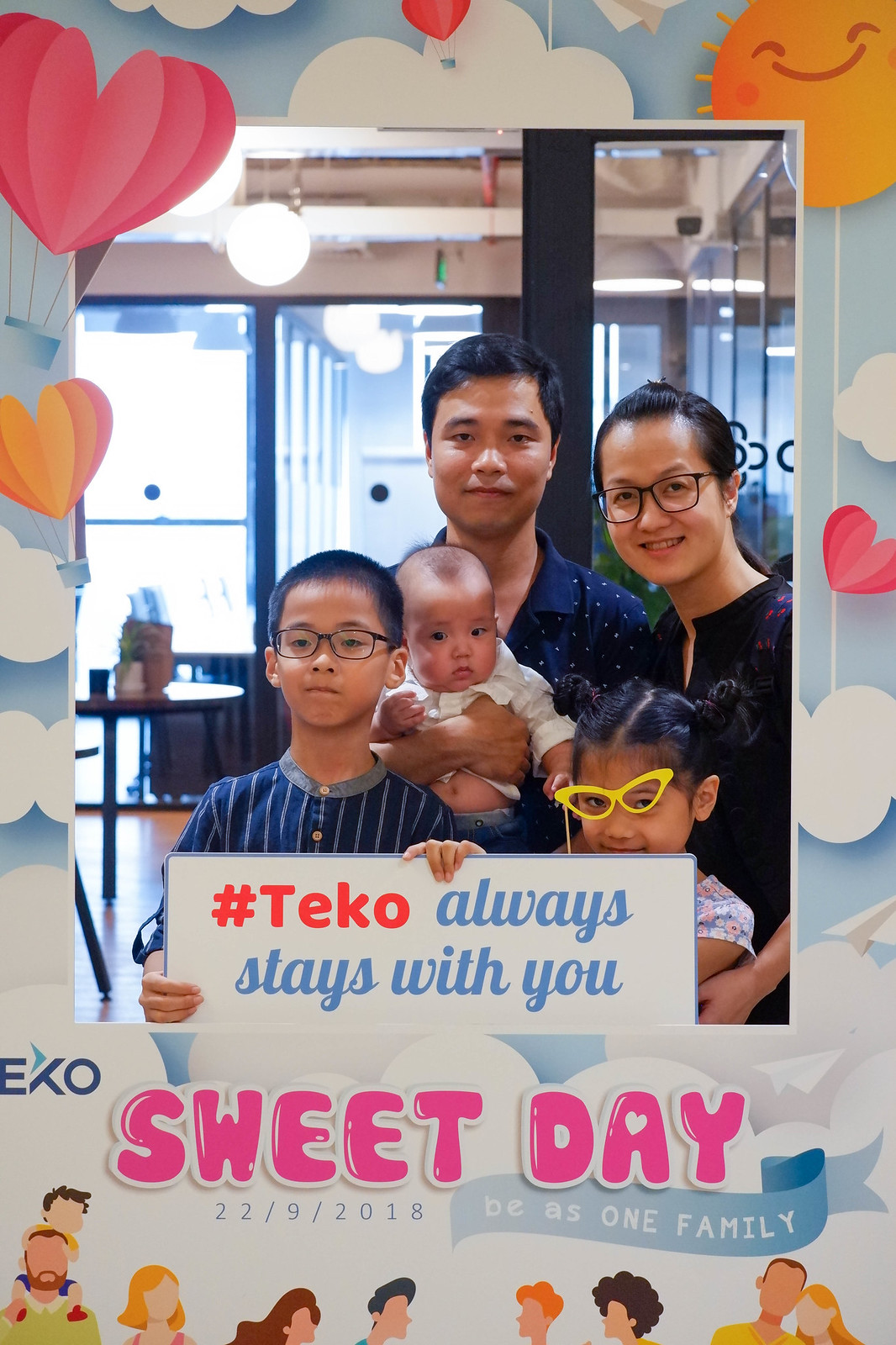The image is a vibrant color photograph, set in a portrait orientation against a decorative border filled with colorful illustrations of hearts, smiling suns, and clouds. The photograph showcases an Asian family standing together, likely in a beautifully lit room with large vertical glass windows in the background. The setting seems to be a restaurant or kitchen, adorned with round tables and chairs. 

In the heart of the image, a man stands smiling, dressed in a dark blue t-shirt and holding a baby wearing a white shirt. Beside him is a young woman with her dark hair tied back and wearing black-rimmed glasses and a black and purple dress. Leaning into the man, she stands on the right side of the photograph. 

In the foreground, a young boy with a crew cut, black-rimmed glasses, and a navy mandarin collar shirt holds a white banner that reads "#TEKO always stays with you," with T.E.K.O. in orange letters. Next to the boy, peeking over the sign, is a small girl wearing funky yellow glasses and with her hair styled like Minnie Mouse. She looks directly at the camera, her playful expression adding charm to the image.

The border of the photograph is detailed with pink, yellow, and white hearts, a smiling sun, and a blue sky with white clouds. At the bottom center, the caption "Sweet Day" is displayed in bold pink balloon-style lettering, followed by the date "22/9/2018" and the phrase "Be as one family" in a blue banner. The lower part of the border also features animated images of adults and children, enhancing the familial and celebratory theme of the image.